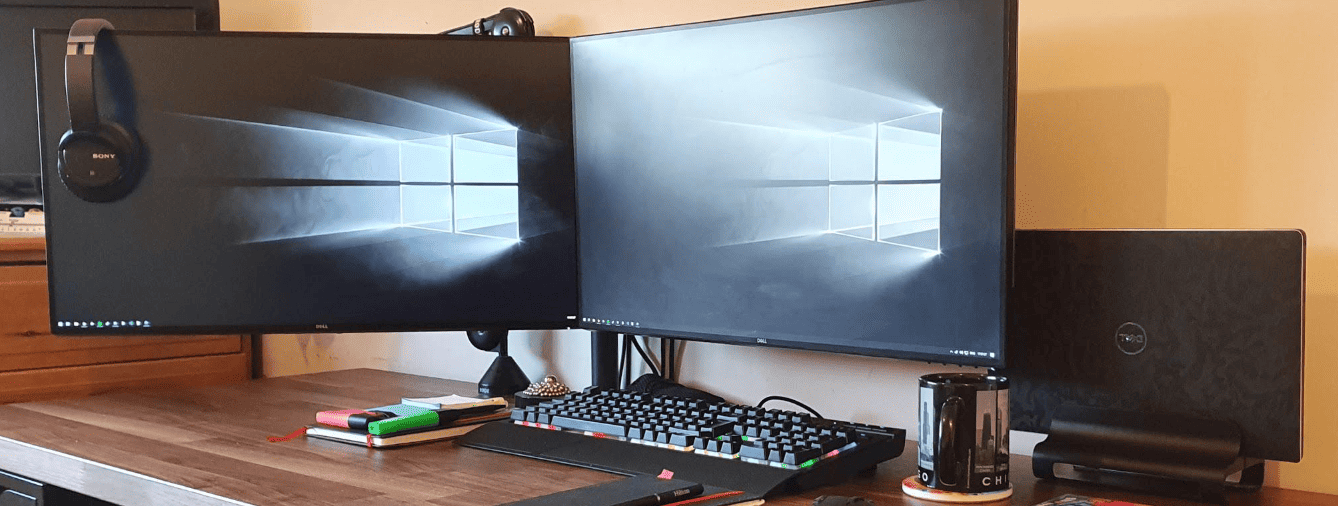This is a detailed color photograph of a person's office desk, showcasing their organized workspace. The desk is made of wood and features a distinctive brown finish with white trim. Prominently displayed are three monitor setups: two larger black monitors, with a pair of headphones resting atop the left monitor, and a smaller, equally tall monitor in the center. The third 'monitor' is actually a Dell laptop on a stand, situated to the right. A reflection of a window emitting light is visible on the screens of the monitors, adding depth to the image.

The desktop itself is black and accompanied by a large black keyboard, whose keys also sport the same dark hue. Scattered across the desk are a couple of markers and some miscellaneous items which blend with the workspace’s professional yet lived-in look. A coffee cup sits atop a coaster on the desk, adding a personal touch to the setup. The wall behind the desk is a warm, inviting orange, contrasting slightly different beige hues previously guessed by others. Additionally, subtle reflections, potentially of a door or more light streaming in, can be seen in the monitor screens, completing the scene of an everyday office environment.